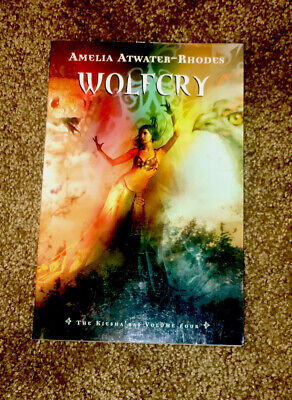In a photograph, a book titled "Wolf Cry" by Amelia Atwater-Rhodes rests on a brown shag carpet. This paperback, part of The Kiesha'ra Series Volume 4, features a vividly colorful cover. Dominating the center of the cover is the image of a woman dressed in a bikini-style top and a skirt, reminiscent of belly dancing attire, with her arms outstretched towards the sky. She appears to be emerging from a backdrop of green trees, with vibrant hues radiating around her: red and orange on the left and yellow on the right. Flanking her, the fiery, glowing colors merge into the red and golden outlines of a snake’s head on the left and an eagle’s head on the right. At the bottom of the cover, dark, shrub-like shapes are faintly visible, adding to the mystical feel of the artwork.